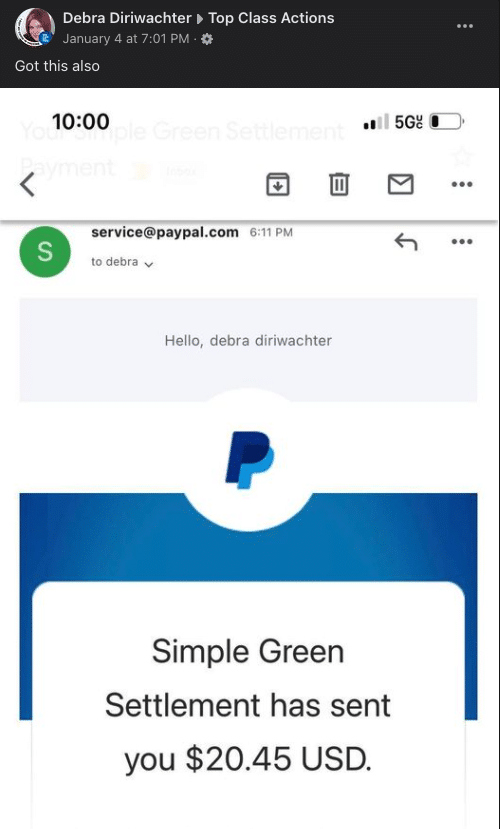Here is a detailed and cleaned-up caption for the image described:

---

The email from PayPal features a sleek black header at the top. Prominently displayed within a circular image is a photograph of a woman with burgundy hair. To the right of the image, in bold white text, the name "Deborah Iriwachter" is displayed, with an arrowhead icon filled in gray pointing to the right beside it, accompanied by the text "Top Class Actions." Further to the right, three vertical dots indicate additional options.

Below this section, in small gray text, is the date and time, "January 4 at 7:01 PM," followed by a bullet point and a light gray gear icon. The main content of the email begins with the text "Got this also," written in white.

Beneath this header is a screenshot from an iPhone, showing the device status bar at the top. It displays a bold black "10:00" on the top left, indicating the time. To the right, the status bar shows a signal strength of two out of four bars, "5G UC" connectivity, and a battery icon indicating about 25% charge.

In the main view of the screenshot, a navigation arrow pointing left is located on the left side of the screen. This is followed by a three-dimensional-looking square icon with a downward-pointing gray arrow on its face, a delete icon represented by a trash can, an envelope icon, and finally, three vertical gray dots on the far right.

Centrally positioned within the screenshot is the classic PayPal logo, standing out against a white background.